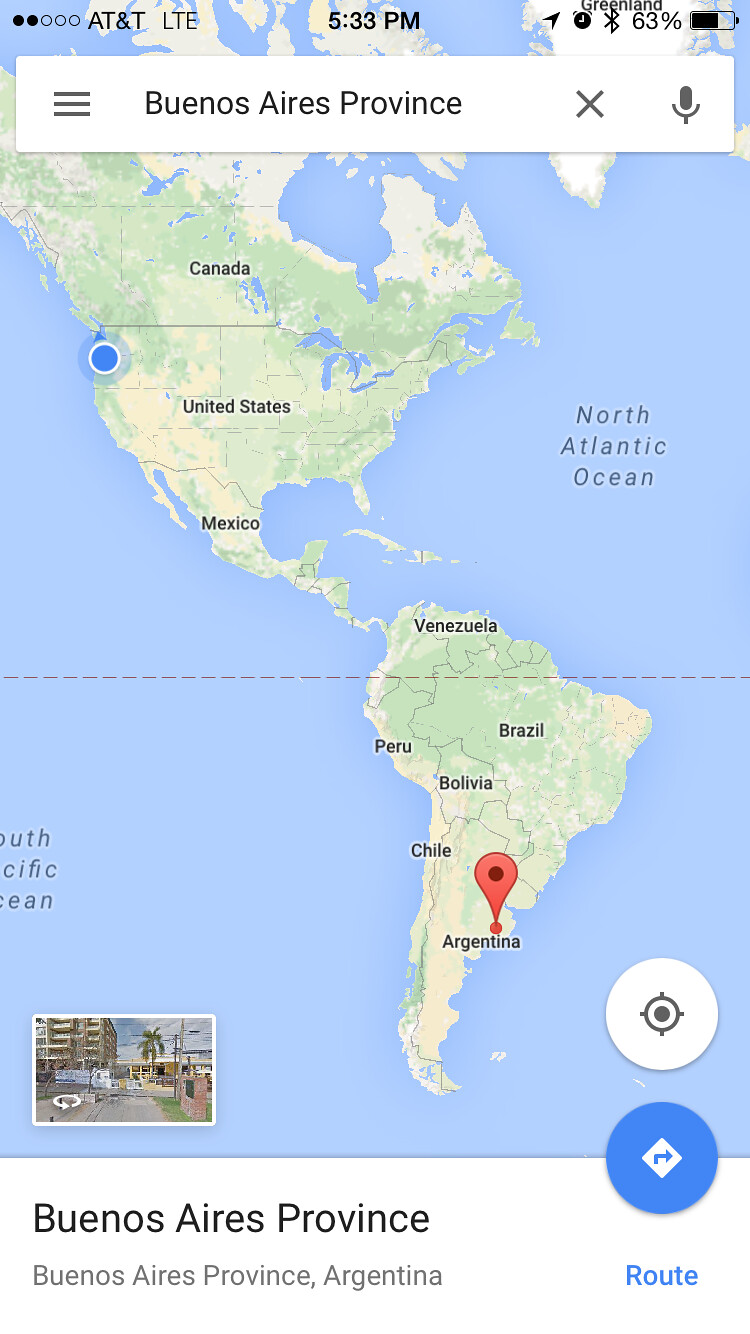This is a detailed screenshot of a smartphone screen displaying a world map, focusing on the Buenos Aires Province in Argentina. The map spans from the Arctic Circle to the southern tip of South America and includes parts of the South Pacific and North Atlantic Oceans. A red pin marks the Buenos Aires Province on the map, and the South Atlantic Ocean is prominently visible. You can see the North Atlantic with the outlines of Mexico, the United States, and Canada on the map.

At the bottom left, there's a small thumbnail image, presumably showing a resort area with a large building and a palm tree, which represents the destination. The map also features a round orientation symbol at the bottom right and a blue circle with a right-pointing arrow below it.

The top of the screen displays phone icons: AT&T, LTE, the time (5:33 PM), and the battery level (63%), along with a Bluetooth symbol. There is a white search bar at the top reading "Buenos Aires Province," with an X and a microphone symbol next to it. The routes and various colors—green, blue, red, white, and black—are visible at the bottom of the screen, indicative of different paths and geographical markings.